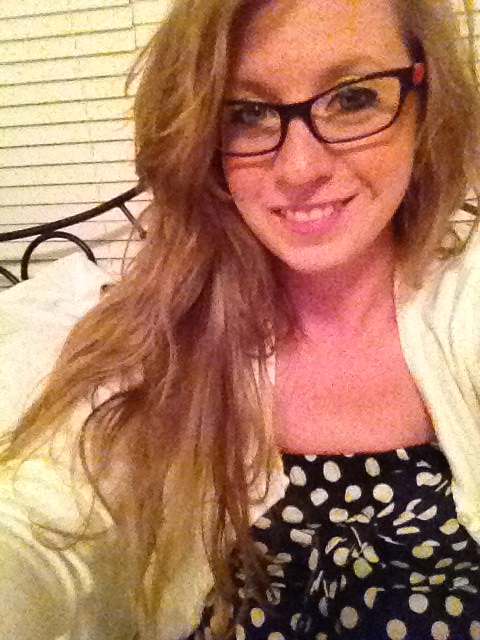This close-up selfie captures a smiling white woman with long brownish hair draped over her right shoulder (from her perspective). Her hair partially covers her left arm, which extends out of the frame beyond her elbow. Her other arm is mostly out of view, with just a hint of her shoulder visible. She wears black-framed glasses and has hazel eyes, her mouth open just enough to reveal the top of her teeth. She is dressed in a light yellow, open jacket over a black dress adorned with yellow and white circles. The scene suggests she is seated on her bed, as a white pillow and a headboard with black bars are visible behind her. Further back, there are closed window blinds, contributing to the cozy, indoor atmosphere of the image.